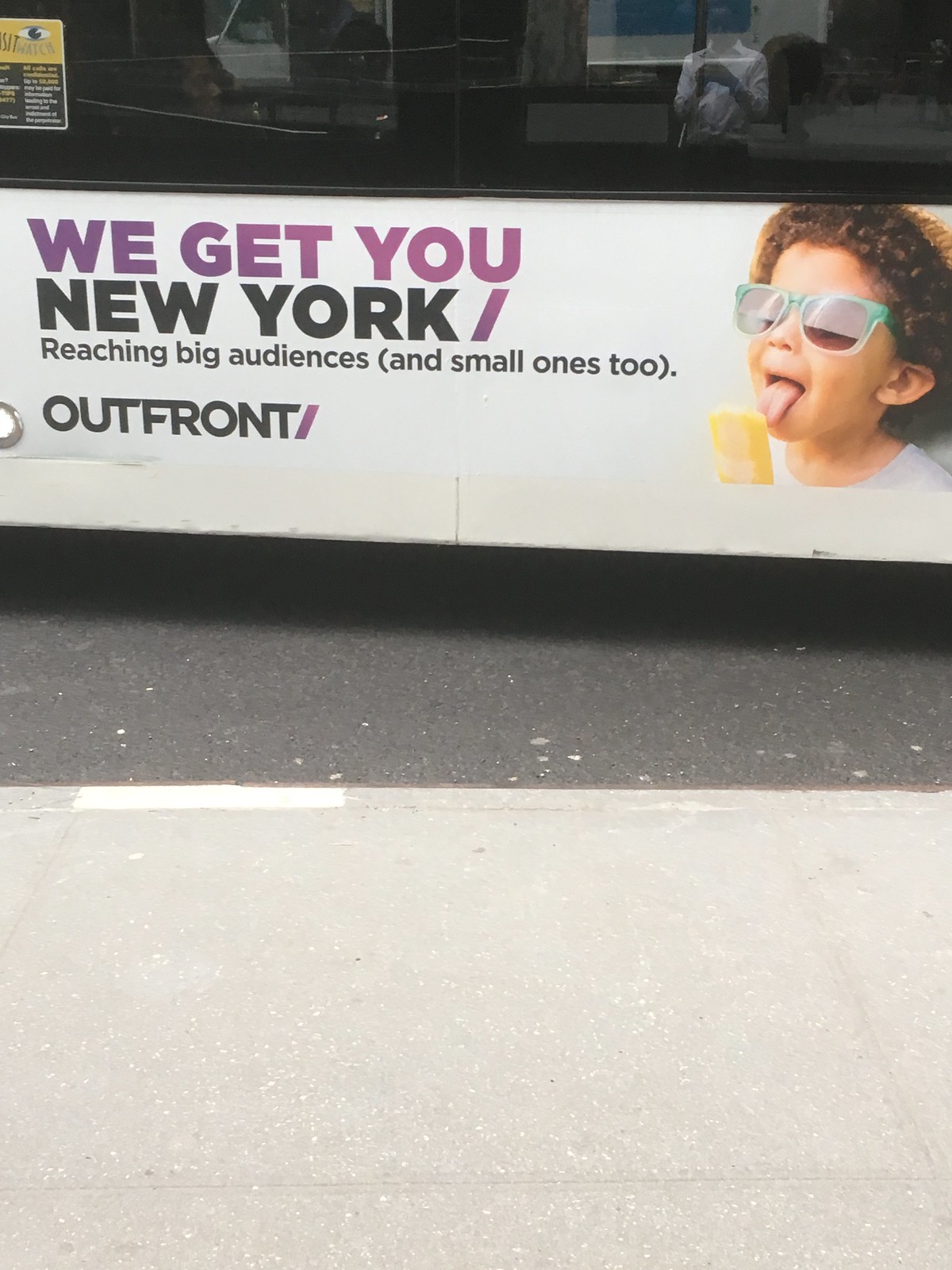This vertical image captures an advertising sign affixed to the side of an unidentified building. Positioned beneath the ledge of a window above, the sign projects outward, almost box-like in its design. The window's glass is notably dark, reflecting a truck and other surrounding objects, adding an urban feel to the scene.

The sign itself is predominantly white, featuring a mix of purplish and black lettering spread over four lines. The topmost line in purple capital letters reads, "We Get You." Below this, in three lines of black text, it says: "New York, reaching big audiences (and small ones too)." 

On the right side of the sign, there is a vibrant image of a young boy with curly hair wearing oversized blue sunglasses, enthusiastically licking a yellow Popsicle. The child is dressed in a simple white crewneck t-shirt, adding an element of casual innocence and delight to the advertisement.